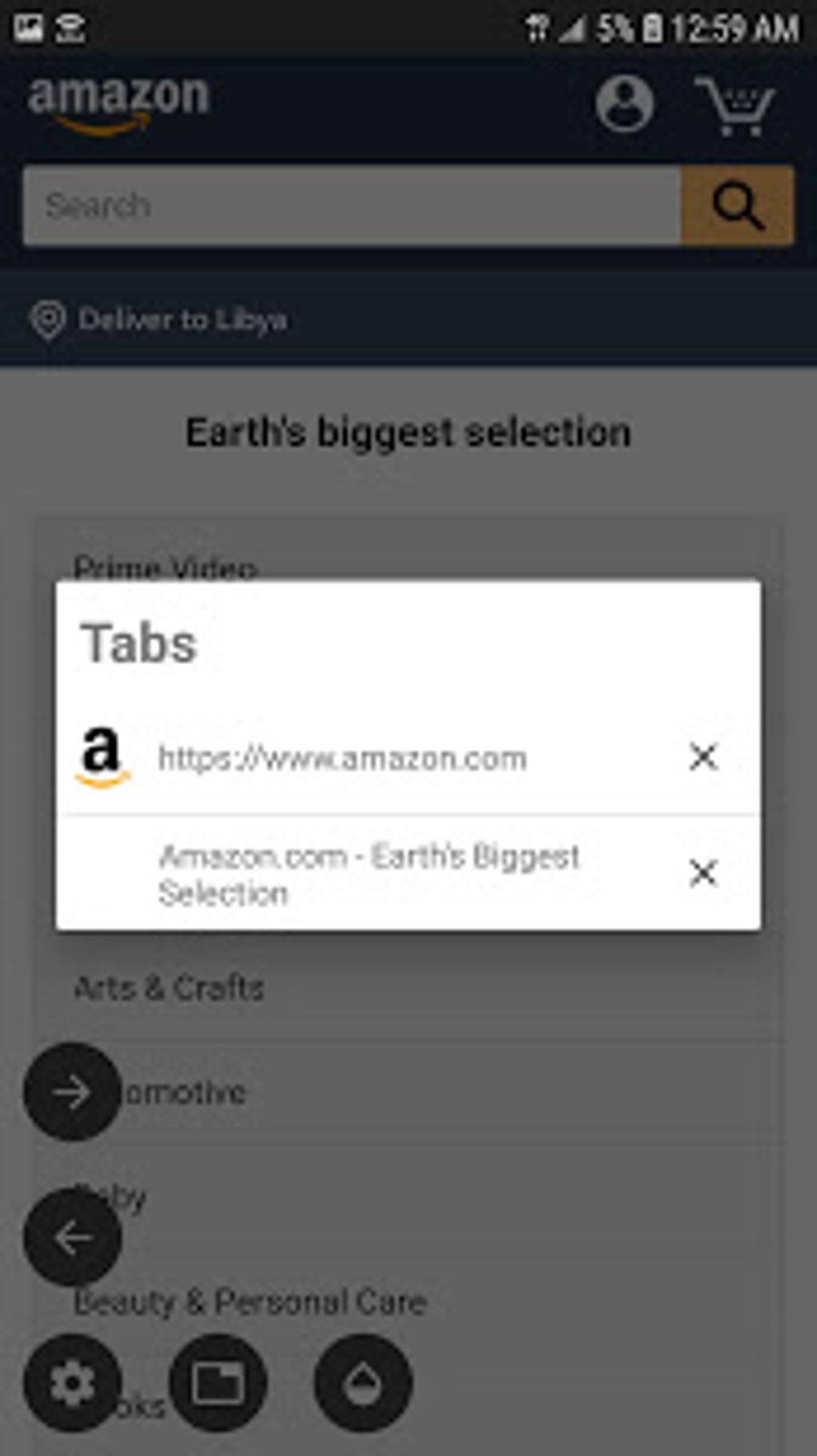This screenshot showcases a mobile device screen displaying multiple browser tabs open in an Amazon shopping app. The screen has been grayed out due to the activation of the tabs button, bringing a white overlay box to the forefront with the heading "Tabs." Within this box, there are two specific tabs listed: one marked with the Amazon logo and URL, "https://www.amazon.com," and the other labeled "amazon.com - Earth's biggest selection," each featuring a closeable "X" icon.

In the background, the semi-visible Amazon homepage provides several elements: at the screen's top left are icons for Wi-Fi and images, while the top right displays the 4G signal strength, a 5% battery life indicator, and the current time, 12:59 AM.

Below these status icons, the Amazon homepage showcases the iconic Amazon logo with an orange arrow forming a smile, and the default user profile picture next to a shopping cart icon. Beneath this is a search bar, complete with a white input area and an orange submit button adorned with a black search icon. Further down, there's a message stating "Deliver to Libya," followed by the tagline "Earth's Biggest Selection."

The visible section of the homepage offers a glimpse of various categories, such as Prime Video and three partially obscured options, along with "Arts and Crafts," "Automotive," and "Beauty and Personal Care."

At the bottom of the screen, there are navigation icons including a right arrow, left arrow, settings, a page icon, and a water droplet icon, facilitating user interaction with the app.